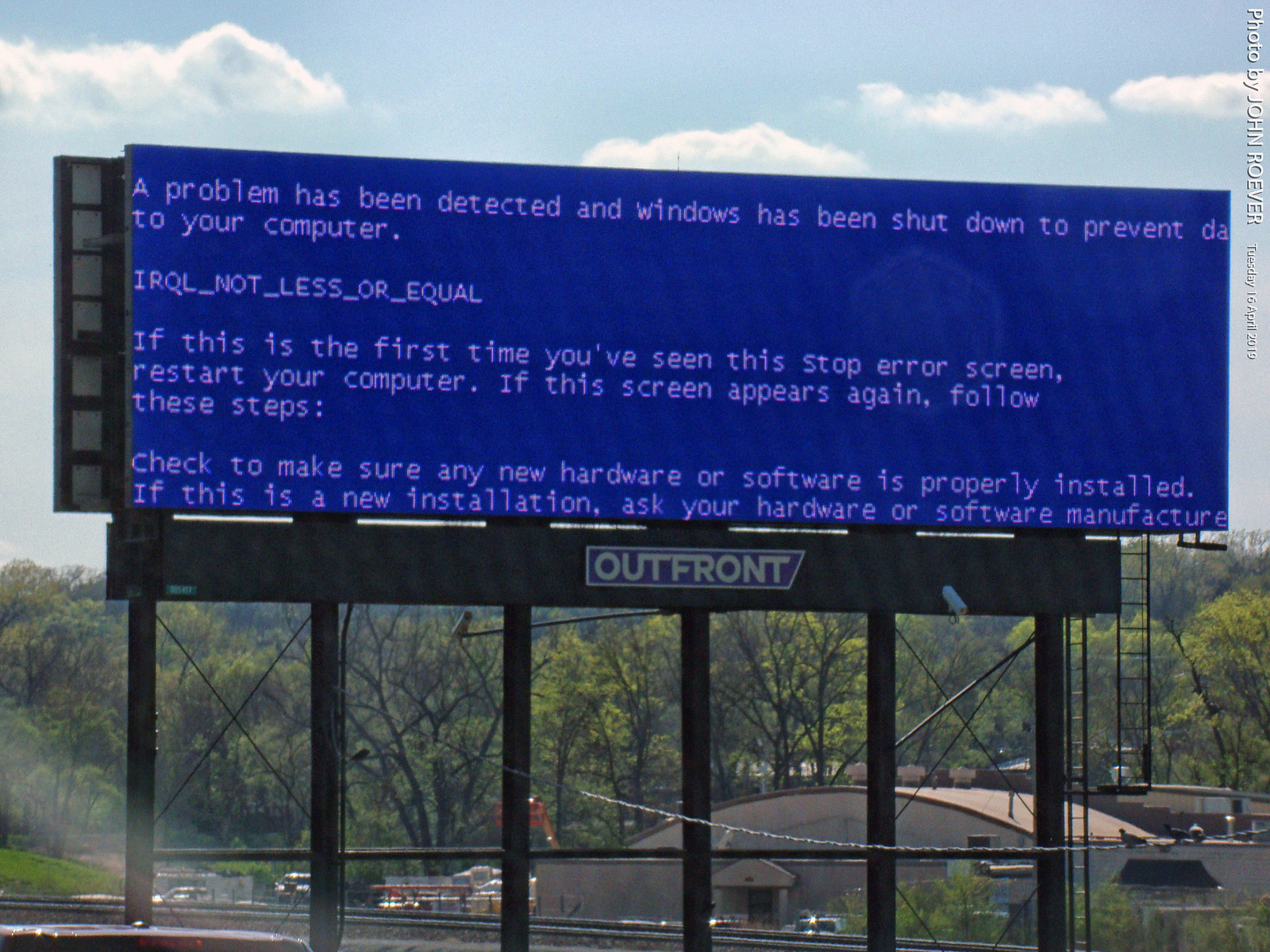The photograph captures a large electronic billboard held up by several slender black metal columns, located outdoors on a bright, clear day. The backdrop features a scenic view with lush green trees and a bright blue sky dotted with fluffy white clouds. The billboard displays a blue screen of death typically seen on Windows computers, with white text warning of a problem and instructing the user on steps to take if the error reappears. The prominent text reads, "A problem has been detected and Windows has been shut down to prevent damage to your computer." The sign visually emphasizes the alarming message against its digital backdrop, making it stand out amidst the natural scenery that includes a round-top building and train tracks below.